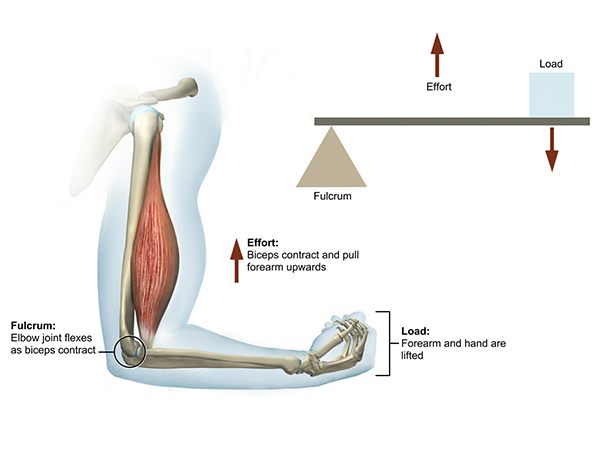The rectangular, white-background informational image depicts an anatomically detailed, hand-drawn arm with transparent skin, revealing the internal bones of the hand, forearm, upper arm, and shoulder, along with partial upper arm muscles. Various sections of the arm are labeled in text. Highlights include: "Fulcrum," with an arrow pointing to the elbow, explaining that the "elbow joint flexes as biceps contract;" "Effort," marked by a red arrow near the upper arm muscle, indicating "biceps contract and pull forearm upwards;" and "Load," directed at the hand, clarifying "forearm and hand are lifted." Additionally, the right part of the image features a diagram with geometric shapes, illustrating movement principles: a long rectangle with a triangle (labeled as "fulcrum") at the bottom left and a square (denoted "load") at the top right, along with arrows signifying "effort." The color scheme consists mainly of brown, black, and oxblood shades.